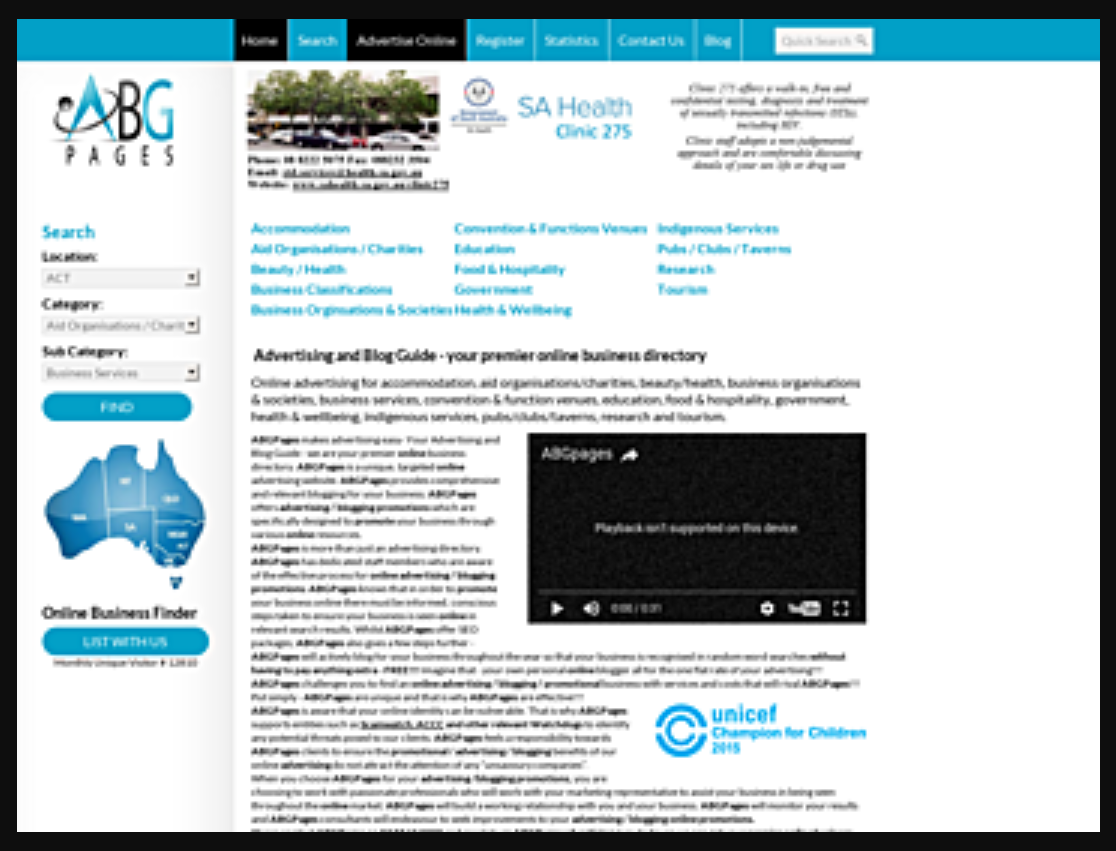This image displays a somewhat blurry screenshot featuring the A, B, and G pages of a website. A prominent blue horizontal menu bar stretches across the top of the page, containing navigation options such as Home, Search, Contact Us, and Blog. To the upper right of this bar is a small search field. 

On the left-hand side of the image, there is a more detailed vertical search section. This section starts with a search field at the top, followed by filters labeled Location, Category, and what appears to be Company. Below the filters, a blue 'Find' button is visible. 

Further down the page, a map showcasing five adjacent states is displayed. Near the map, the phrase "Online Business Finder" appears in black font. Underneath this text, there is another blue button.